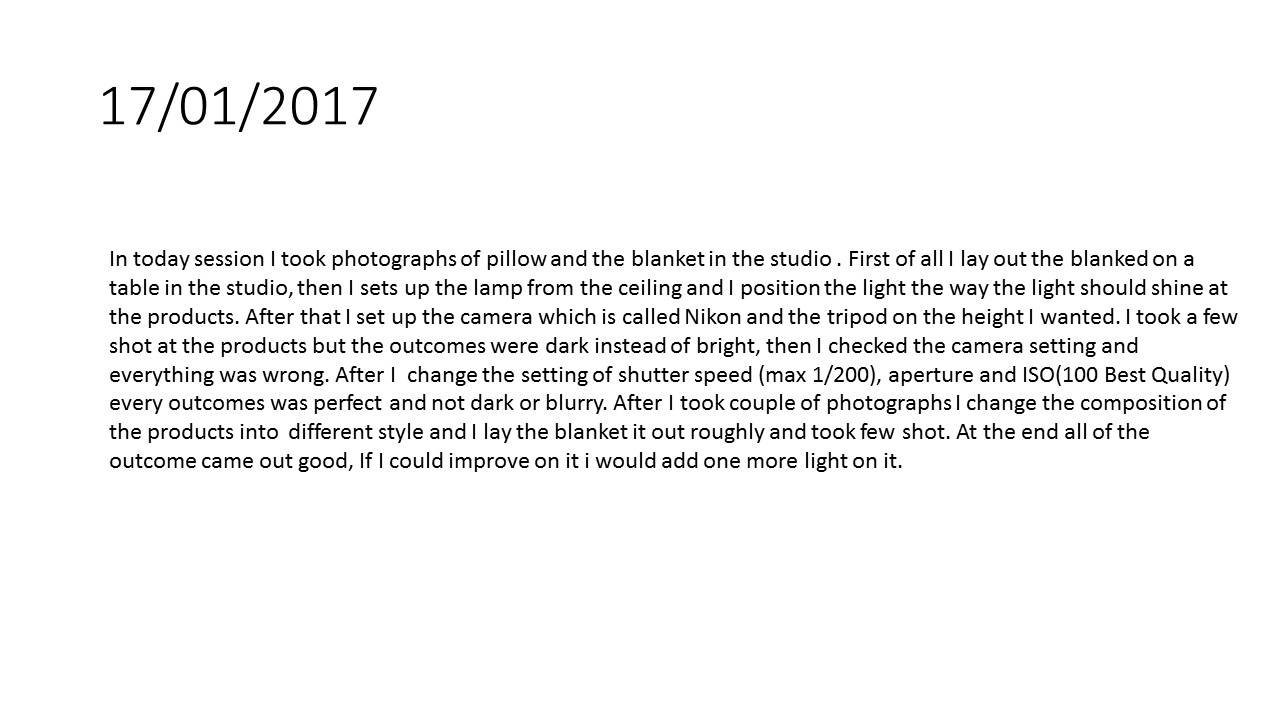The image depicts a scanned document with a white background and black text. In the top left corner, it is dated "17/01/2017". Below the date, a detailed paragraph describes a photography session in a studio. The document outlines the following steps taken during the session: First, the photographer laid out a blanket on a table and set up a ceiling lamp to shine light on the products, which included a pillow and the blanket. Next, the camera, a Nikon, was mounted on a tripod adjusted to the desired height. Initial shots resulted in dark images, prompting the photographer to check and correct the camera settings, including the shutter speed (max 1/200), aperture, and ISO (100, best quality). After adjusting these settings, subsequent photographs came out well-lit and clear. Further adjustments involved rearranging the composition of the products and taking additional shots, all of which turned out satisfactory. The photographer noted that adding one more light could improve the setup. This entry appears part of a photo journal detailing the studio photography process and adjustments.